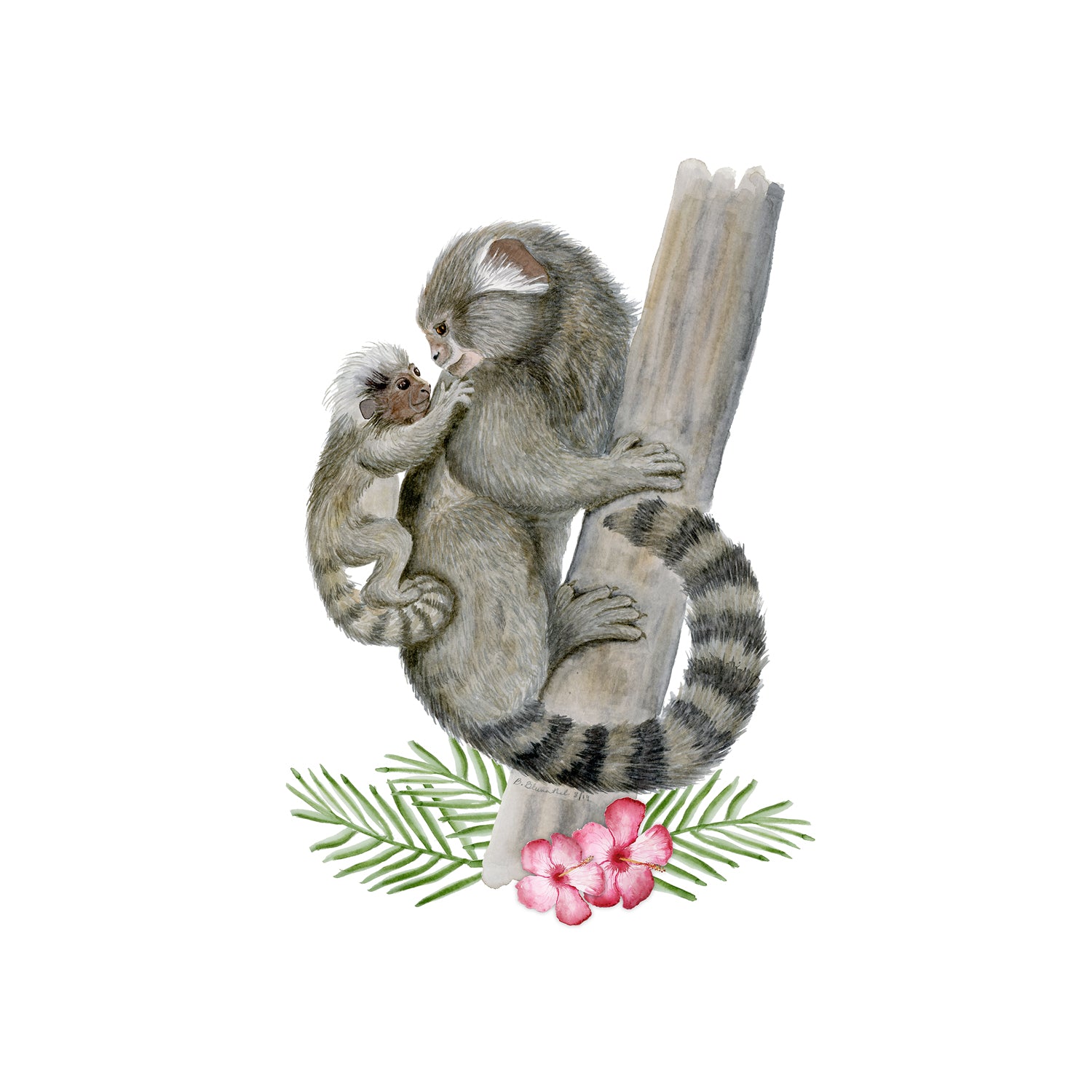This detailed drawing depicts a tree trunk with two vibrant pink flowers, each bordered with red and surrounded by three green leaves, positioned at the bottom. Ascending the tree is a gray primate, perhaps a lemur or monkey, characterized by a raccoon-like tail marked with black and gray stripes. The mother, with her short, narrow face and white ears, is captured looking back affectionately at her baby, holding onto her shoulders. The baby, also gray with a less defined striped tail and a white head, mirrors this gaze, adding a touch of warmth to the scene. Both figures exhibit subtle smiles, infusing the image with a tender, familial connection. The tree stretches vertically across a white background, slightly angling to the right at the top, situating the subjects within a naturally vivid setting.